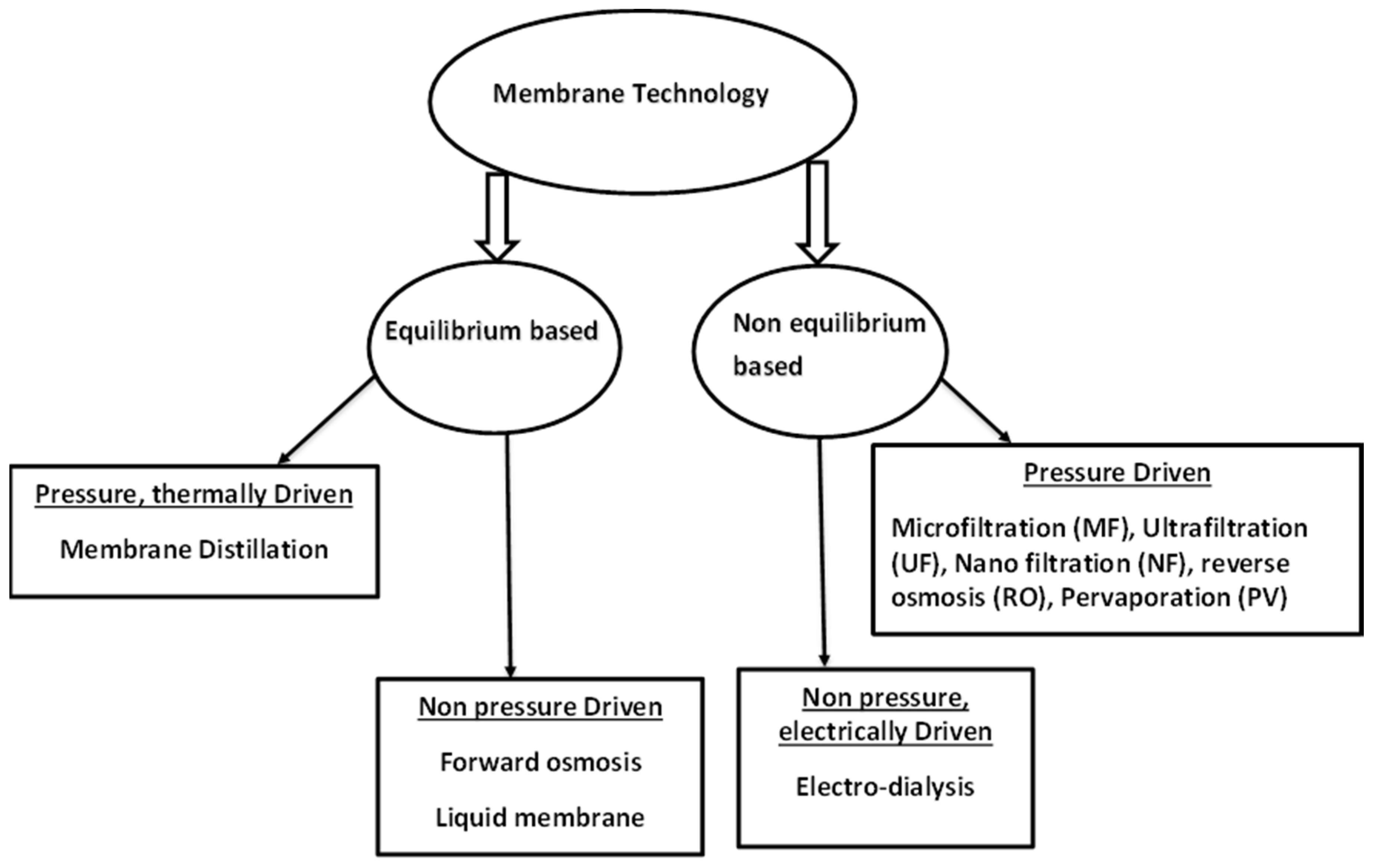The image is a detailed informational flowchart delineating different types of membrane technology. At the top, there is a black-outlined oval with a white background containing the text "Membrane Technology" in black font. Two arrows, white-outlined in black, point downwards from this oval, leading to two smaller ovals: "Equilibrium Based" on the left and "Non-Equilibrium Based" on the right. Both ovals have black font text and thin black line arrows extending downwards.

Under "Equilibrium Based," two rectangles are positioned sequentially downward. The first rectangle is labeled "Pressure Thermally Driven," which is underlined, followed by "Membrane Distillation." The second rectangle, connected by another downward arrow, reads "Non-Pressure Driven," also underlined, with "Forward Osmosis Liquid Membrane" beneath it.

Under "Non-Equilibrium Based," there are also two rectangular boxes. The first rectangle to the left says "Non-Pressure Electrically Driven" with "Electrodialysis" beneath it. To the right, the second rectangle is labeled "Pressure Driven" and lists multiple processes: "Microfiltration (MF)," "Ultrafiltration (UF)," "Nanofiltration (NF)," "Reverse Osmosis (RO)," and "Pervaporation (PV)." 

This comprehensive diagram categorizes various membrane technologies based on equilibrium principles and driving factors.